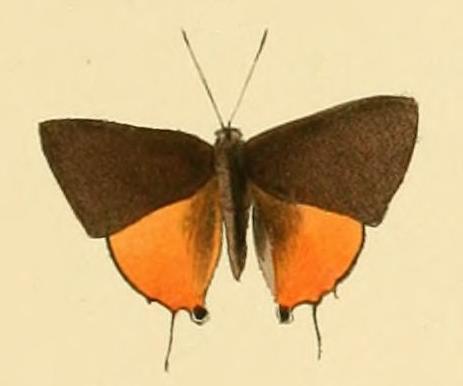The image captures a detailed illustration of a moth or butterfly, centered against a light beige paper background that resembles parchment. The insect is presented from above, showcasing its two distinct pairs of wings. The upper wings are a rich brown, while the lower wings are a lighter orange with brown shading, featuring two black tail-like extensions at the bottom. The body of the moth is a brown color, similar to the upper wings, and it is positioned prominently in the center of the image. The insect has two thin antennas extending from its head, pointing outward. The style of the artwork is akin to an illustrative watercolor, often found in botanical manuals or insect species guides. The orange wings appear semi-transparent, possibly suggesting an illusion of wings underneath, adding to the delicate, intricate nature of the drawing.